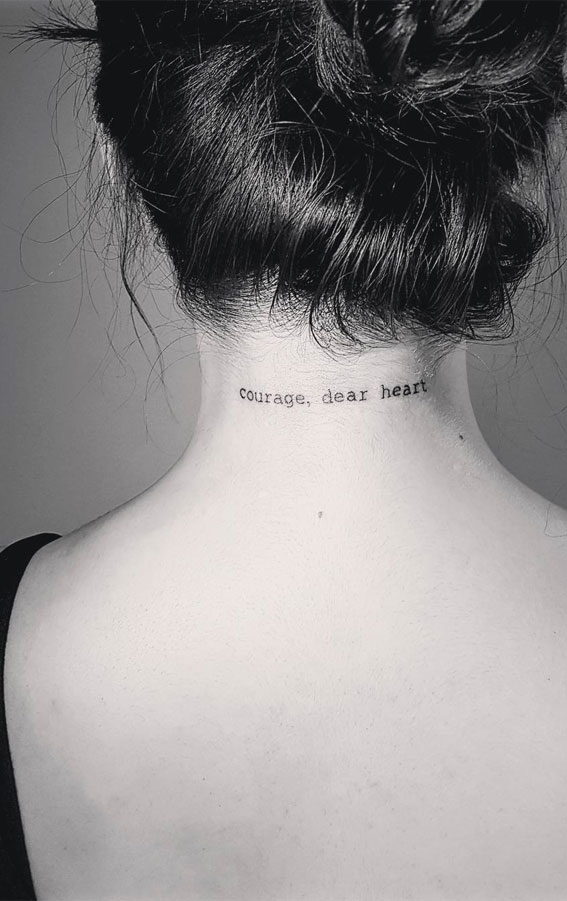This black-and-white photograph captures the back view of a woman, focusing on her upper back and neck, with the top of her head also visible. Her dark hair is styled in a loose, wavy bun with stray strands hanging down. On the back of her neck, there is a tattoo with the words "courage, dear heart" written in all lowercase letters. She is wearing a black tank top, identifiable by a visible black strap on her left shoulder. The right strap is not seen due to the image's angle and cropping. Additionally, a prominent black mole is visible on the right side of her neck near the tattoo, and a couple of smaller moles can be seen on her back. The background is blank, making the woman the central focus of the image.